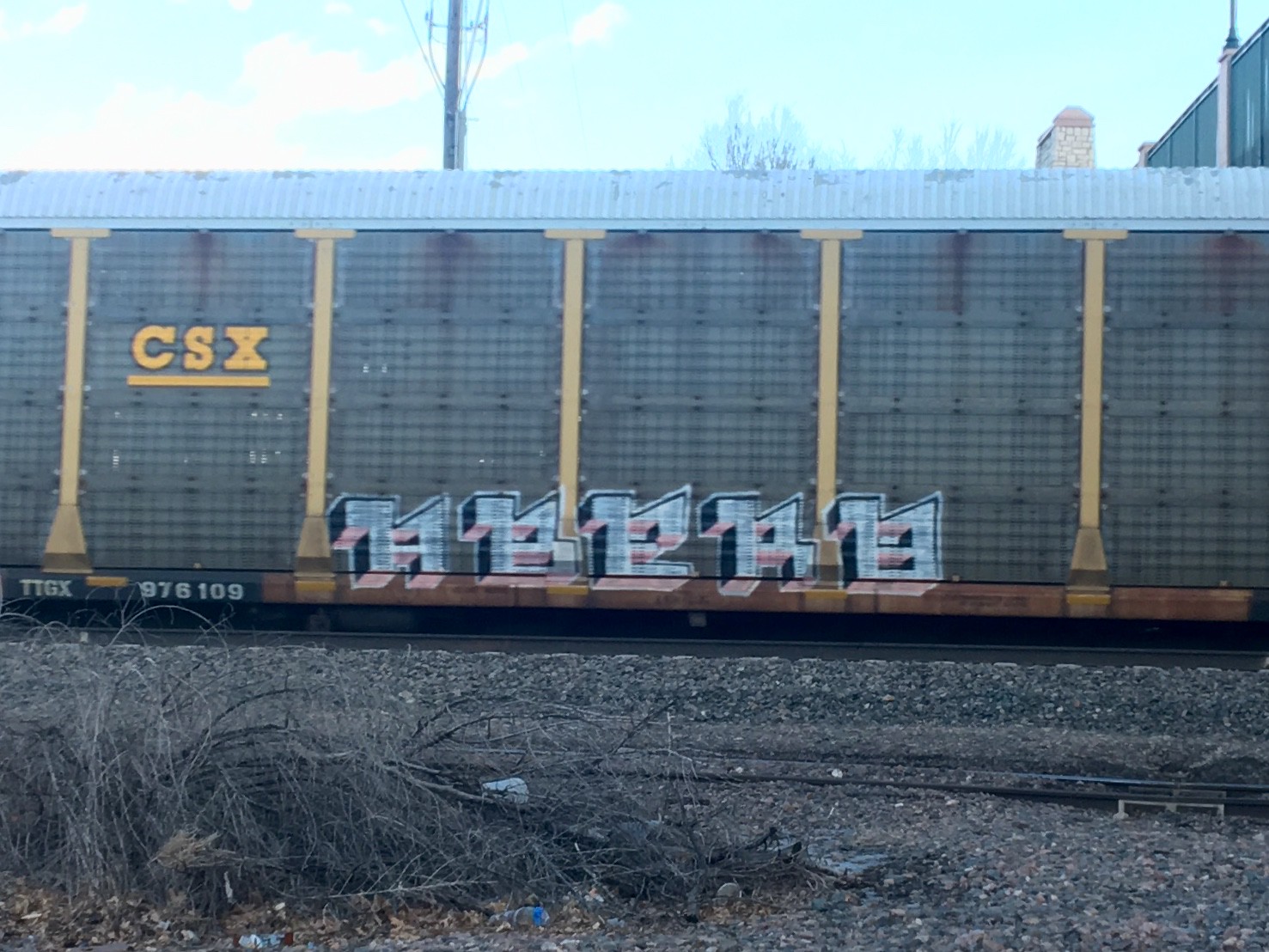The photograph showcases a weathered train car positioned on a gravel-covered track during winter. The large, enclosed container is prominently labeled with the CSX logo in yellow on the far left, while faded graffiti in a foreign script adorns the center of the carriage. The container is brown with a silver roof, and five subdividing metal rails, some of which are yellow, accentuate its surface. Detailed inscriptions at the base include TIGX and the numbers 976109. The surroundings feature dormant grass and bush, with a telephone pole and a distant building in the background, all under a blue, lightly clouded sky.